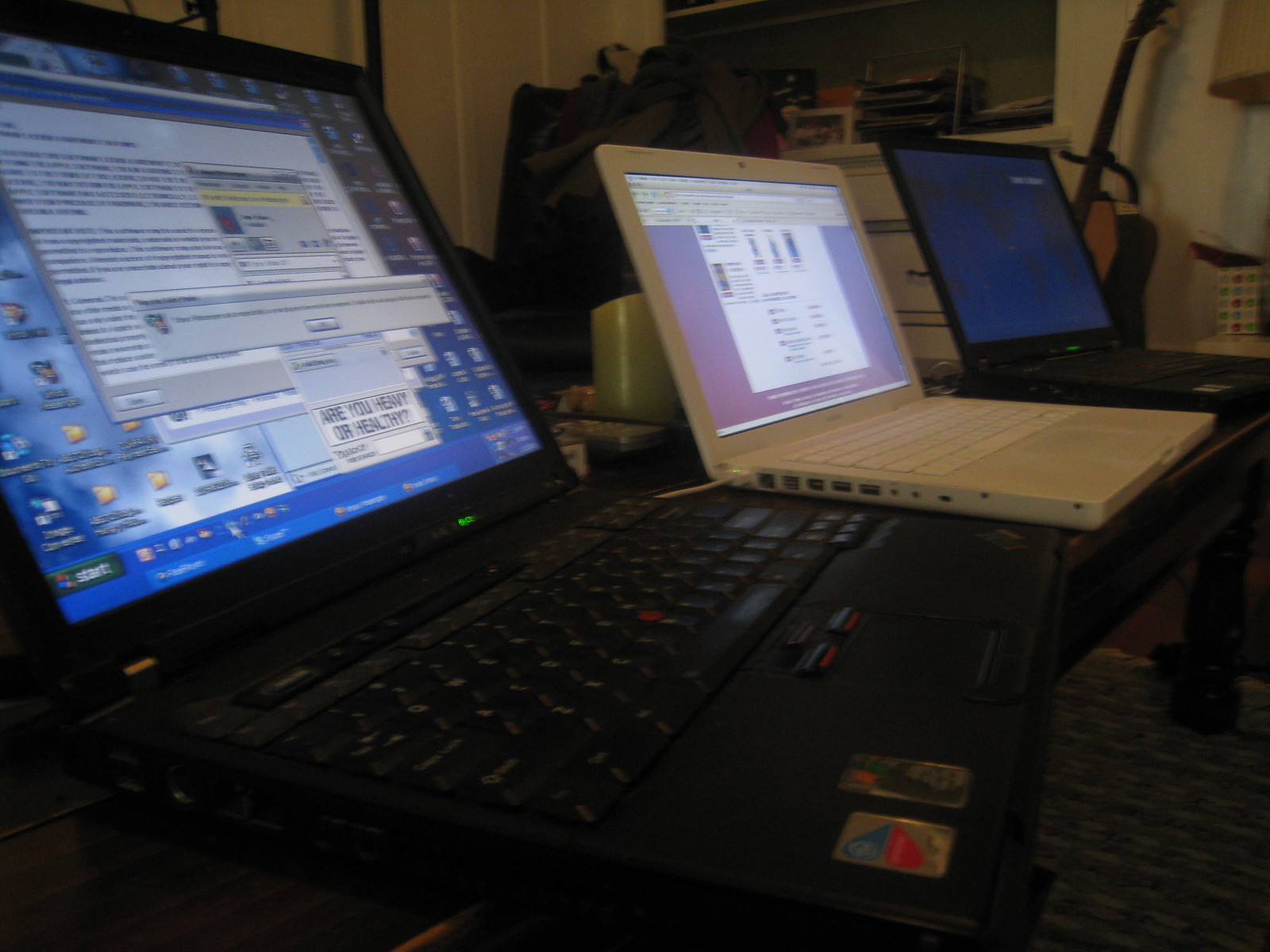The image depicts a cluttered, possibly makeshift workspace or home setting with three different open laptops lined up on what appears to be a low wooden coffee table, under which lies a woven rug. The laptop in the center is an older, light beige plastic model, possibly an old MacBook, while the ones on either side are more standard dark grey or black. All three appear to be running Windows; the outer two have blue home screens. The screen of the laptop closest to us displays some blurry text with a pop-up message, including the text "Are you heavy or healthy?" The central beige laptop shows a window with a purple background and a white box containing text and images, though the details are unclear. The third laptop has a blue screen that might be a desktop image of a world map. The background reveals a guitar on a stand, partially obscured by the laptops, and a chair draped with clothes. Additionally, there's a green candle and shelving units or racks filled with various items, contributing to the overall impression of a crowded and disorganized space. The lighting is poor, adding to the image's sense of messiness and dated quality.